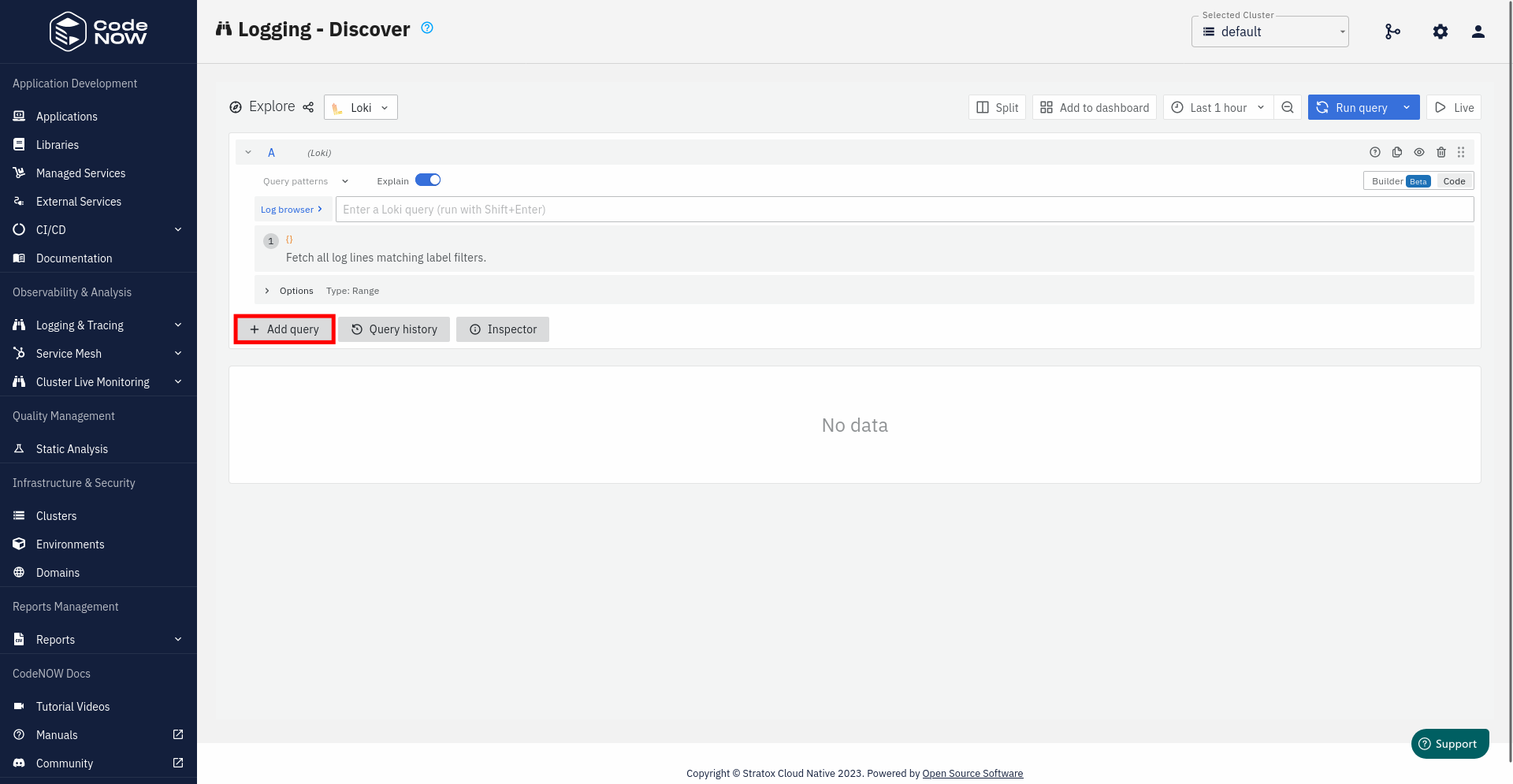The image features a user interface on a gray background. The interface displays a central section with a cube icon signifying code, accompanied by an ongoing log labeled "discover." To the right of this section are two icons: one for settings, and another for user profile, adjacent to an "explore" option.

A prominent gray bar spans across the interface, beneath which lie two larger gray rectangles, followed by three smaller ones. The first of these smaller rectangles is marked "add query" with a plus sign, highlighted by a red outline. Below this, two additional small rectangles are labeled "query history" and "inspector."

A white rectangle, positioned lower in the interface, indicates "no data" in gray text. Finally, at the bottom of the interface, a green oval resembling a power button is present, emblazoned with the word "support."